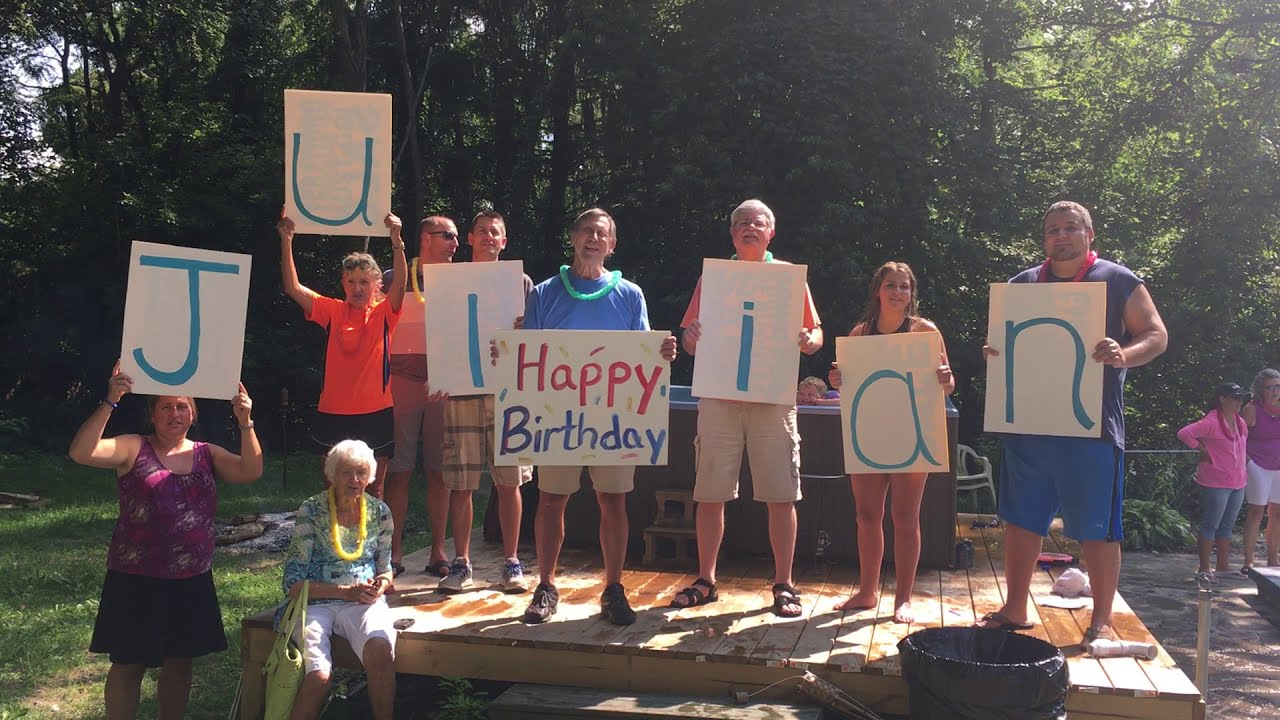In the image, a group of individuals are gathered on a wooden deck platform, celebrating a birthday. This diverse group, ranging in age from children to elderly, is likely a family enjoying a summer day outdoors. Each person is holding a white poster board with a handwritten letter on it, collectively spelling out "J-U-L-I-A-N." Notably, one poster in the middle says "Happy Birthday" with "Happy" in red text and "Birthday" in blue. 

The individuals are casually dressed, with the lady holding the letter J wearing a purple tank top and black skirt, while the one holding the U sports an orange shirt with dark shorts. The man with the N stands near a trash can lined with a black garbage bag. The platform appears to extend from the front to the back of the image. Surrounding the wooden deck is a lush scene with trees, hinting at a yard backed by a forest.

In the background, some people are near what seems to be a small pool or hot tub, adding to the festive atmosphere. An elderly woman, adorned with a yellow lei, sits in the front center wearing white shorts and a blue blouse, reinforcing the warm summery context of this cheerful celebration.